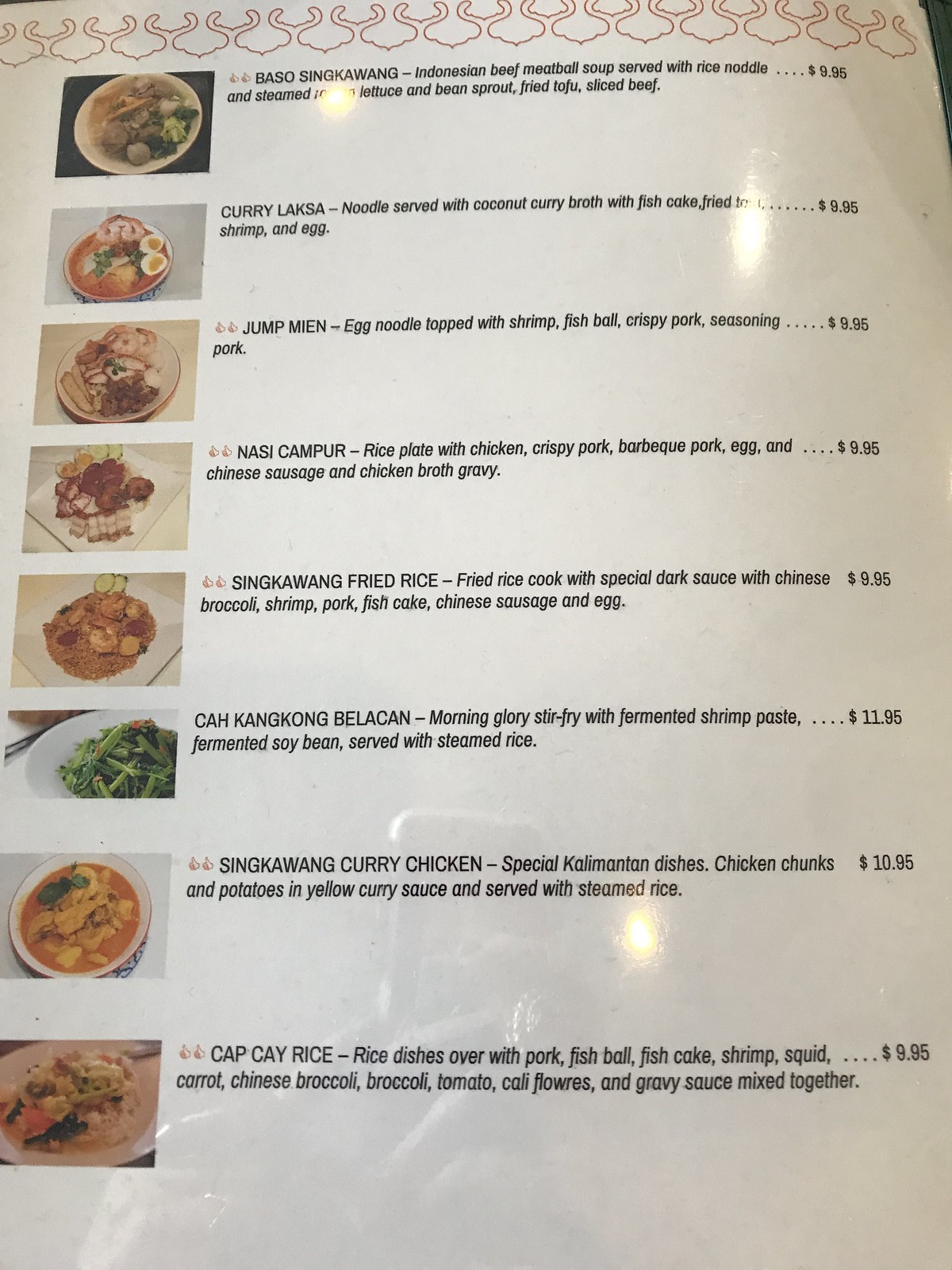This photograph captures a menu inside a restaurant, likely taken by a patron. The menu is the central focus, adorned with a plastic protective covering that produces reflections of ceiling lights and the hand holding a smartphone to snap the picture. The menu presents a series of about eight different dishes, each accompanied by a small photograph on the left, depicting the dish's appearance.

To the right of each dish's name and description, the prices are clearly listed. Among the offerings are various rice dishes and curries. Notable items include:

- **Curry Laksa**: Noodles served with coconut curry broth, fish cake, fried tofu, shrimp, and egg, priced at $9.95.
- **Jump Me In**: Egg noodles topped with shrimp, fish ball, crispy pork, and seasoned pork, also priced at $9.95.
- **Baso Sengkawang**: An Indonesian beef meatball soup.

The detailed layout and vivid descriptions make it easy for patrons to decide on their meal choices.